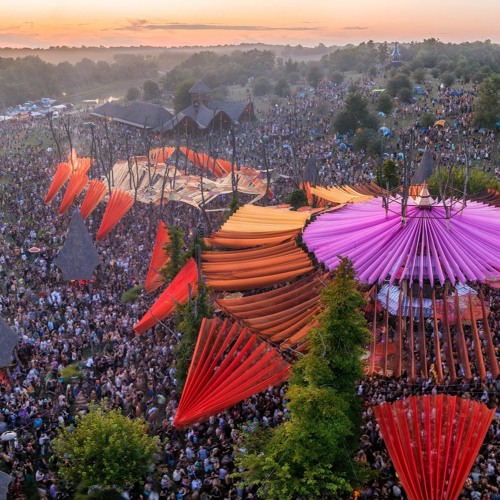This is an aerial photograph capturing a bustling outdoor fairground filled with people, tents, and various structures. Prominent in the image are two large tent-like structures: one on the right, which is notably purple and yellow, and another on the left, which is primarily beige. Both are surrounded by smaller tents in shades of beige, red, and orange. Scattered trees dot the area, becoming denser towards the horizon. In the background, towards the front, cars and buildings are visible. The sky overhead displays a gradient of orange and yellow hues, adding a warm, vibrant atmosphere to the scene. The ground area is packed with attendees, suggesting the event, possibly a concert or fair, is highly attended.